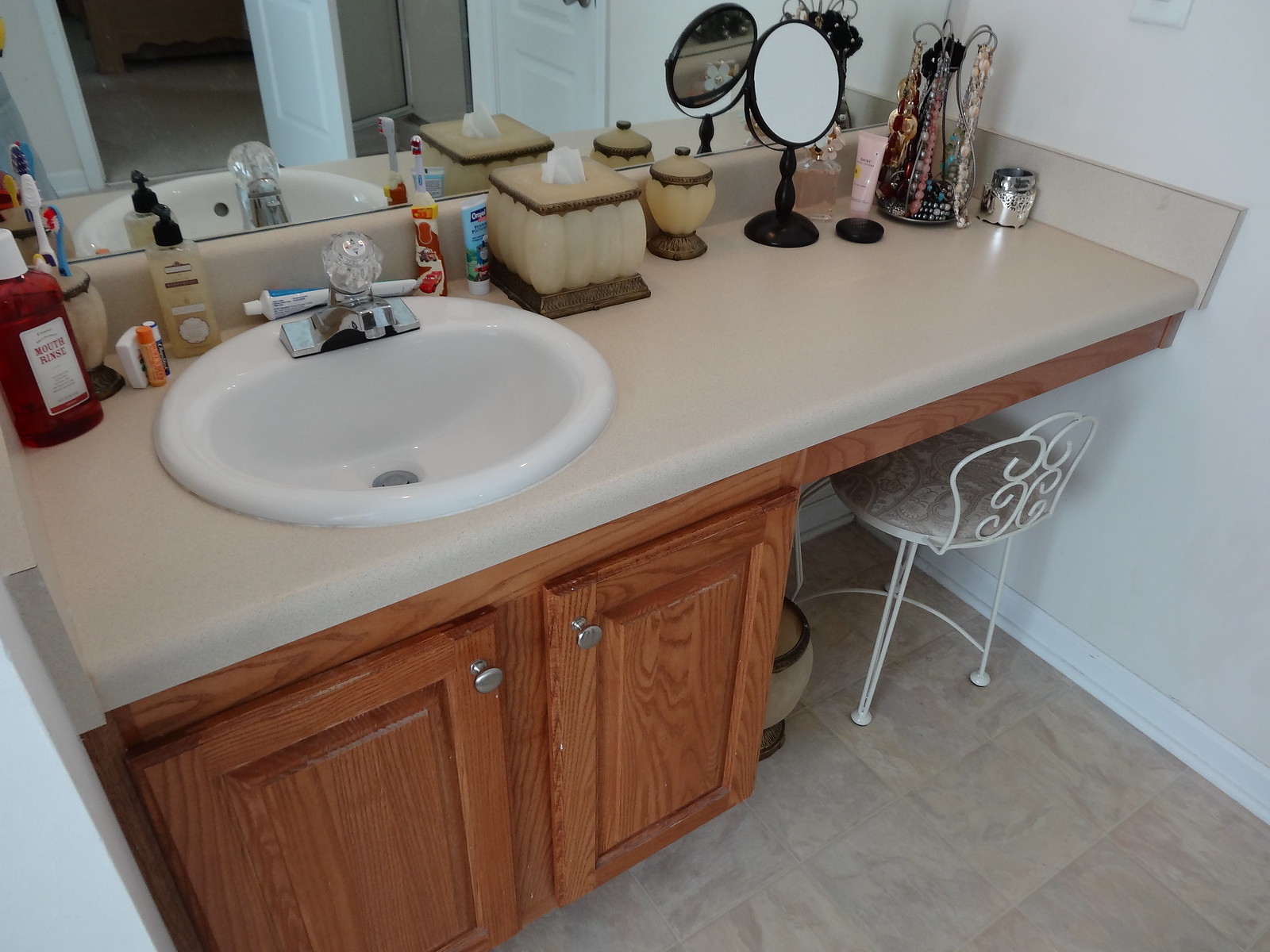This landscape-oriented photo captures a well-organized bathroom countertop. The counter is a beige-colored surface with a white, round sink fitted with a silver faucet. The countertop is supported by cabinetry fashioned from fabricated oak, featuring silver knobs and two cabinets below. On the right side, the counter transitions into a vanity area with a small, white wrought-iron chair tucked underneath.

The countertop is arrayed with various personal care items, meticulously arranged. A red container labeled "mouthwash" stands prominently. Nearby, a stand holds several toothbrushes alongside a chapstick, dental floss, soap, toothpaste, electric toothbrush, an additional toothpaste, and a tissue dispenser. There is also a small container with a lid, a dark close-up mirror, a pink bottle of perfume, a makeup compact, a small pink lotion bottle, and a stand adorned with assorted necklaces and bracelets. Completing the array is a silver-lidded container.

Below the counter, a matching trash can is visible, harmonizing with the silver-lidded container, tissue holder, and toothbrush holder on the countertop. Together, these elements create a cohesive and functional bathroom vanity space.